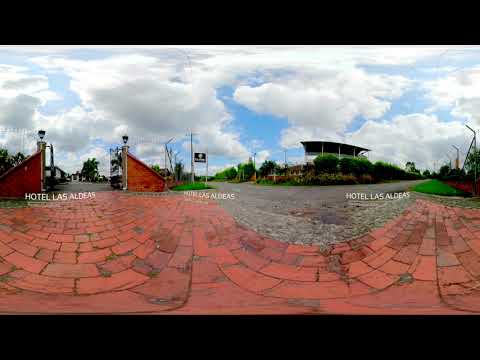The image features a red brick or cobblestone pavement that appears aged and slightly worn, with weeds sprouting between the pavers. The shot seems to have a panoramic style that causes the ground to appear curved. The upper half of the image is dominated by a vibrant blue sky filled with large white and gray clouds. The pavement splits into two directions. On the left side, partially visible brick walls lead to an open gate adorned with lanterns, labeled "Hotel Las Aldeas." Beyond the gate, there are structures that resemble houses or possibly parts of the hotel, alongside some trees that might include palm trees. On the right side of the image, a road diverges in two directions with grass flanking either side and additional buildings visible in the distance. A stand or structure seems to overlook what might be a recreational field. Across the middle of the image, the words "Hotel Las Aldeas" are repeated in white text overlay, serving as a clear advertisement for the location.